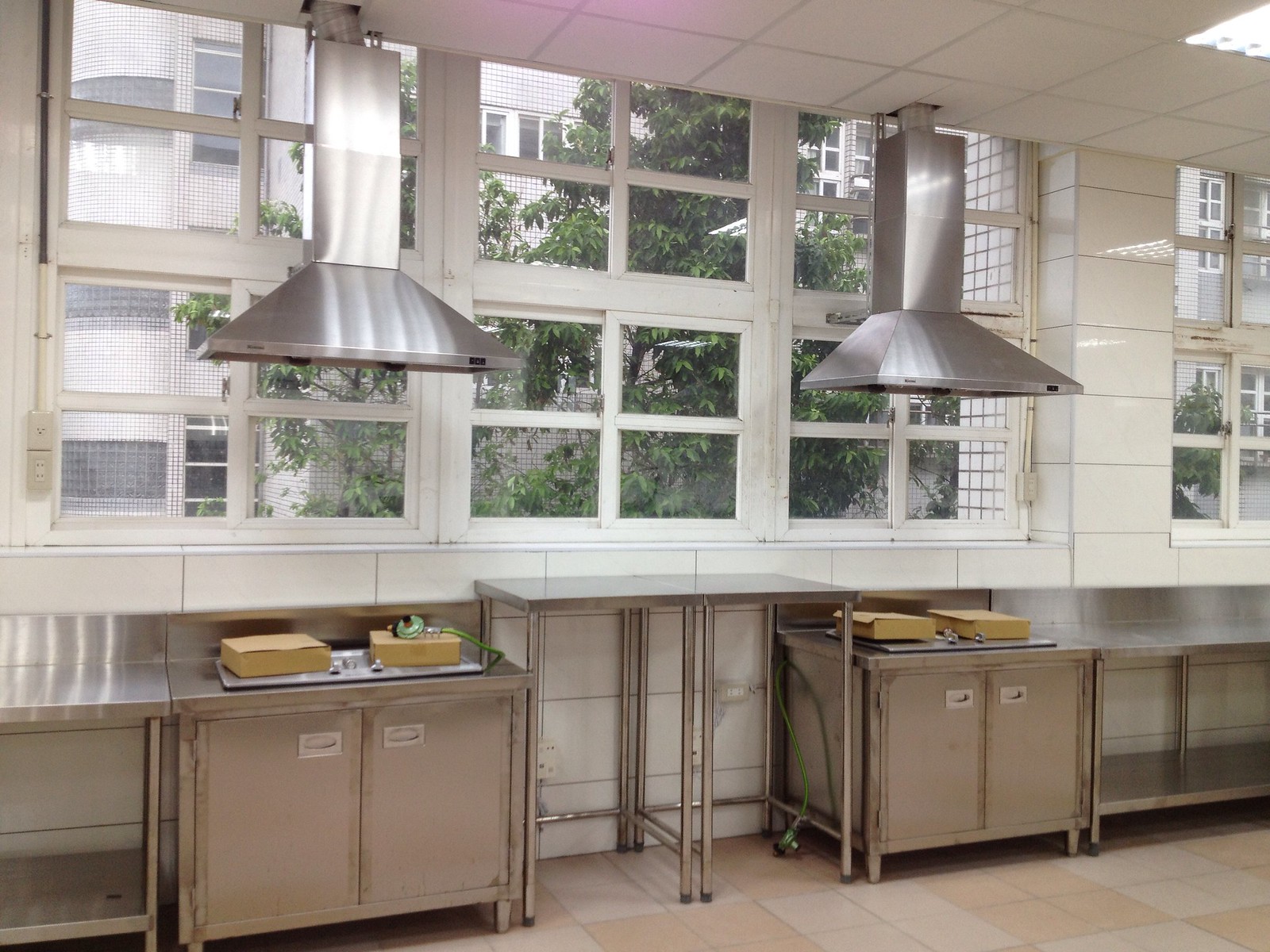This photograph depicts the interior of an industrial kitchen. The room features large, rectangular windows at the top, each divided into eight panes of glass. Outside, you can see green trees and a high-rise white building with numerous windows, indicating a bright daytime setting. Inside, the walls are covered with white tiles, while the floors are lined with beige and cream rectangular tiles. 

Beneath the windows, there are stainless steel countertops and several stainless steel carts with doors that open. On these carts, two brown round objects rest on a silver tray, with boxes stacked beside them. To the side of the carts extends a long stainless steel countertop with two levels. Additionally, two large aluminum vent hoods, designed for exhaust, protrude from the ceiling above the serving carts, reminiscent of those typically found above stoves in commercial kitchen settings.